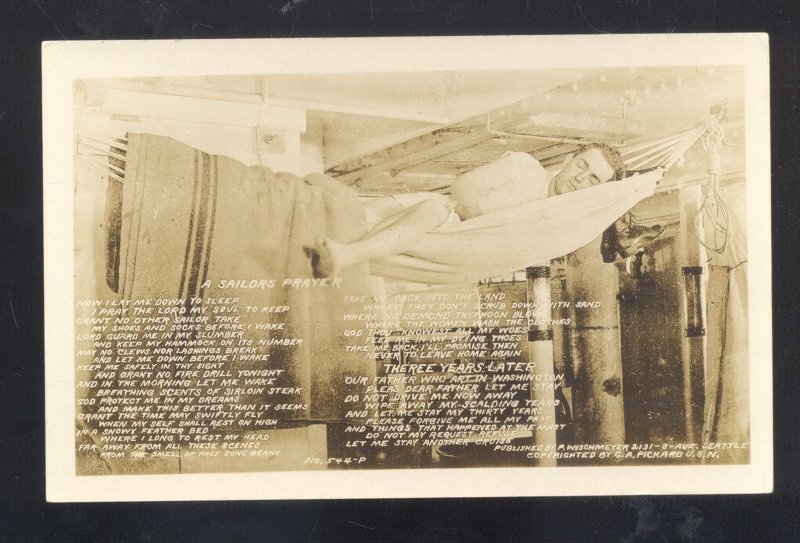In this faded vintage photograph, a sailor is seen resting in a white hammock suspended from the metal ceiling and piping below deck in a ship. The image has a bronze-like hue, lending it a nostalgic, antique feel. The sailor, whose body dominates the upper portion of the frame, is tucked under a blanket. Surrounding him, the ship’s interior is visible, complete with metal walls, rivets on the ceiling, and various pipes. A small lamp and a hung rug can also be discerned in the background.

The photograph is framed with a black border approximately two inches wide. The image itself is on a light tan or beige background. Inscribed on the image in small, white text is "A sailor's prayer," followed by several paragraphs of text, though the exact words are too small to read. Notably, the text overlaps the blanket covering the sailor.

In the bottom right corner, the picture is marked with the credits "Published by P. Wissenmeier, 231 8th Avenue, Seattle" and "Copyright by G.A. Picard, USN, US Navy."